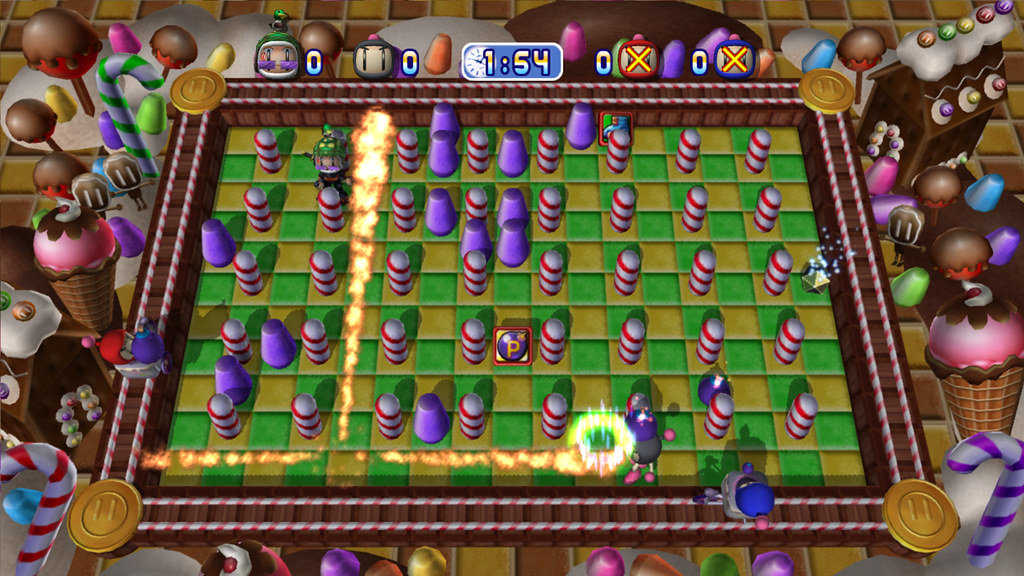This is a screenshot from a candy-themed video game, portraying a dynamic, colorful game board at the center. The game board itself is depicted with green and yellow checkerboard patterns. Vibrant candies surround the board, including red and purple candy canes, red lollipops with chocolate dripping, and strawberry ice cream cones with chocolate ganache. Gumdrops in various colors accentuate the candy landscape. A dark brown gingerbread house adorned with a rainbow of candies is visible in the upper corners.

Within the game board, the play involves making patterns, as suggested by a fireball effect seen moving vertically and horizontally, indicating a match being cleared. Cylindrical candy pieces in red, white, and purple populate the board, with one section actively showing yellow flames, suggesting player action. At the top of the screen, game interface elements display a timer reading 1:54 and other score indicators marked by zeros and an X. The entire scene is vibrant, with each candy and game element drawn in a playful, cartoon style.